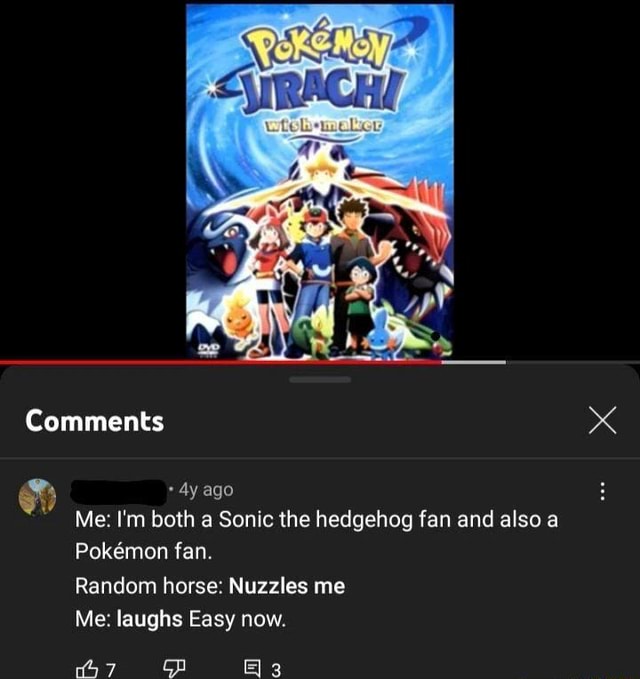The screenshot from YouTube showcases a video currently playing about 75% through, featuring the Pokémon movie "Jirachi: Wishmaker." The DVD cover prominently displayed in the center of the screen is set against a black background. The cover is primarily blue, with vibrant, glittering stars enhancing the overall design. At the bottom center of the cover, various characters from the movie are depicted, including the main character Ash and his iconic companion Pikachu. These characters, along with others, are outlined in white. The title "Pokémon" is displayed in bold yellow letters with a blue outline, while "Jirachi" is written in blue with a white outline, and "Wishmaker" is in yellow with a white outline beneath it.

The comments box at the bottom of the screen shows that a user posted a comment four years ago, expressing their dual fandom for both Sonic the Hedgehog and Pokémon, humorously mentioning a random horse nuzzling them, which elicited laughter. The comment has garnered seven upvotes and three replies.